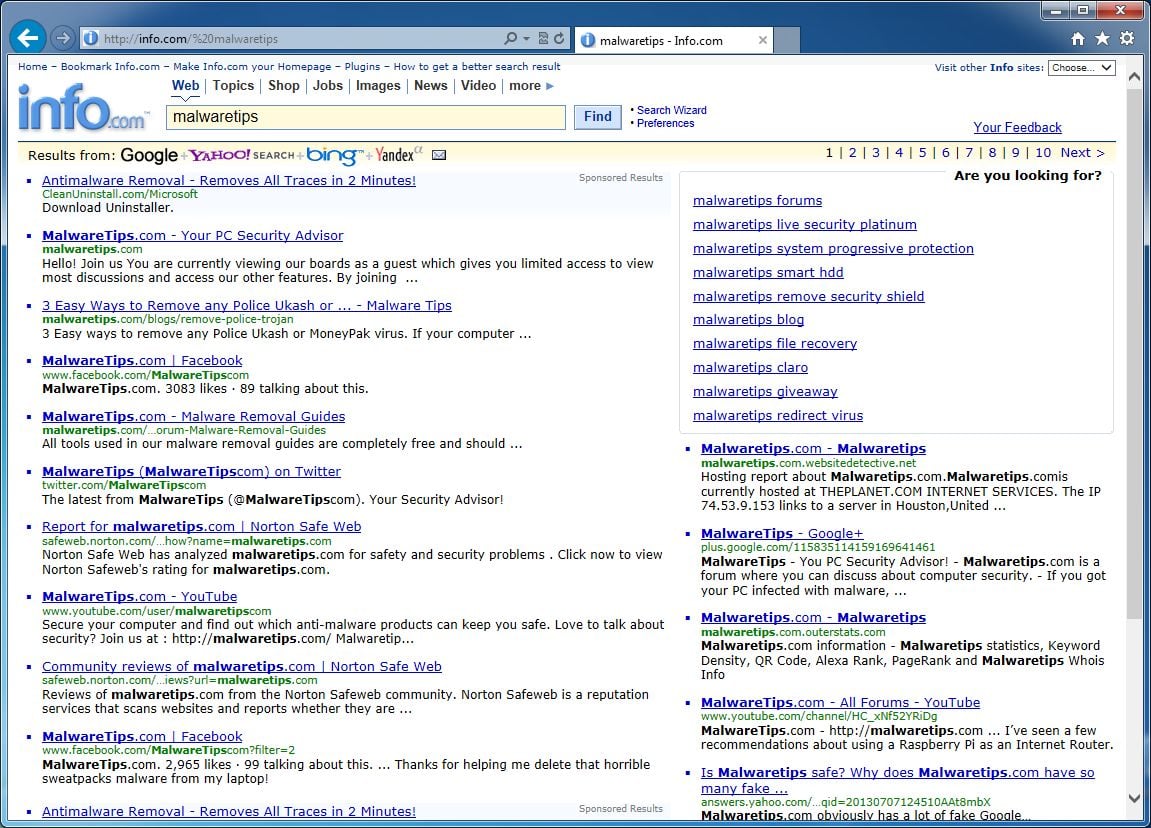The screenshot displays the info.com website with a dark blue border in the top left corner. On the upper left side, there's a white arrow encircled in blue, pointing left, accompanied by a right-pointing arrow beside it. In the search bar, the URL reads "http.info.com," followed by a text snippet, "malware tips info.com". Below the search bar, the text "info.com" is repeated, accompanied by the blue info.com logo. The search query entered is "malware tips".

The results displayed below the query indicate that they are sourced from Google, Yahoo, Search, Plus Bing, and Yandex. The first result is an anti-malware removal service that claims to eliminate all traces in two minutes. The second result is "malwaretips.com - your PC security advisor". Following this, the third result lists "three easy ways to remove any police, UCash, or malware tips". The fourth result directs users to "malwaretips.com Facebook". The page continues in a typical search result layout down to the bottom.